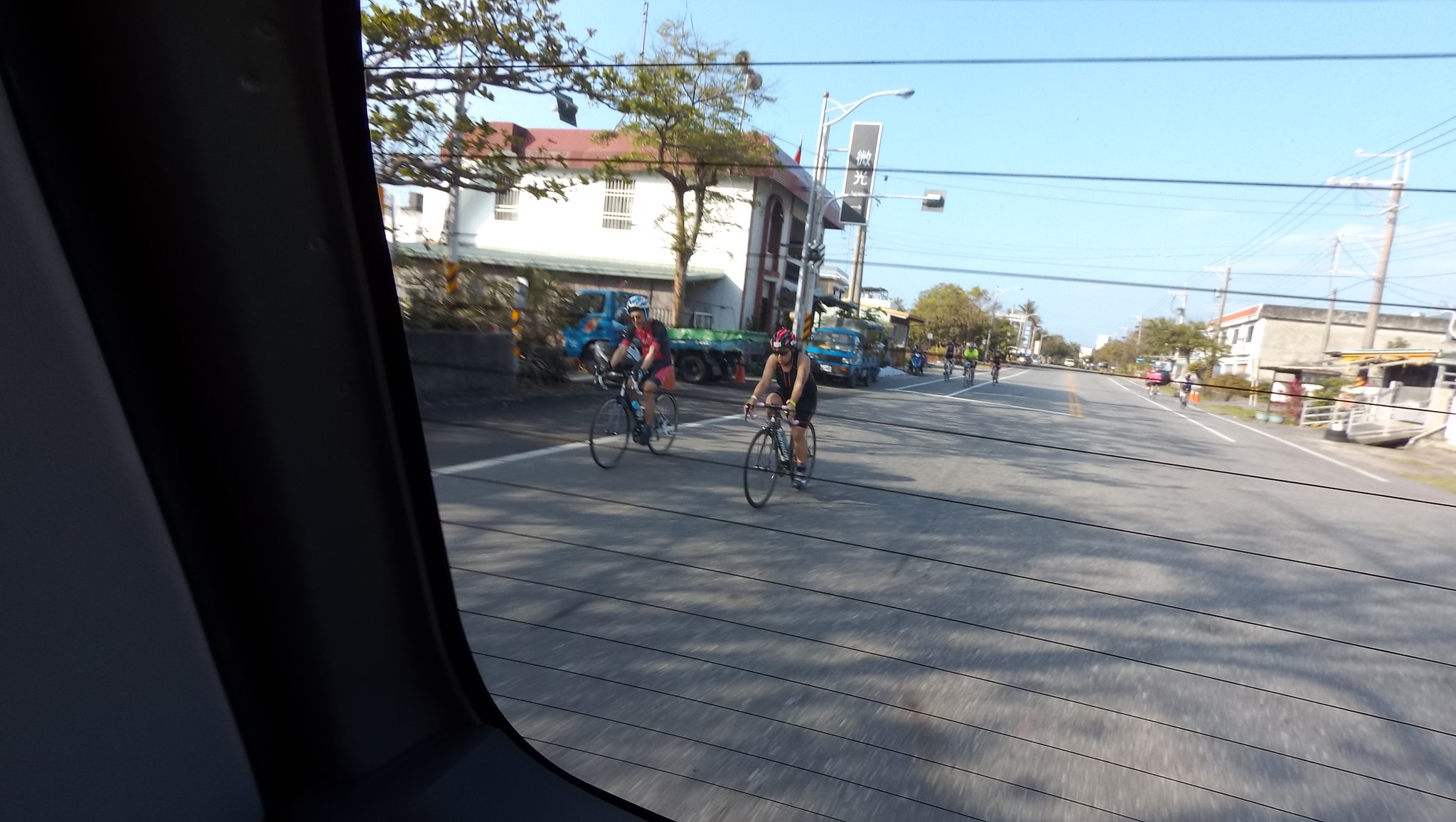This photograph captures a dynamic urban scene through the back windshield of a car. The black defrost lines on the windshield confirm the vantage point. In the foreground, two helmeted cyclists ride race bikes along the side of the road behind the vehicle. The right side of the street features storefronts and various buildings, with the tallest being two stories high. On the left, two blue delivery trucks are parked near a building. Further down the road, more cyclists and pedestrians populate the scene, adding to the bustling atmosphere. The painted lines on the pavement extend halfway down the road, enhancing the sense of depth. Additionally, a portion of the car's interior and the backseat mirror frame the left edge of the image, emphasizing the viewer's perspective from inside the vehicle.